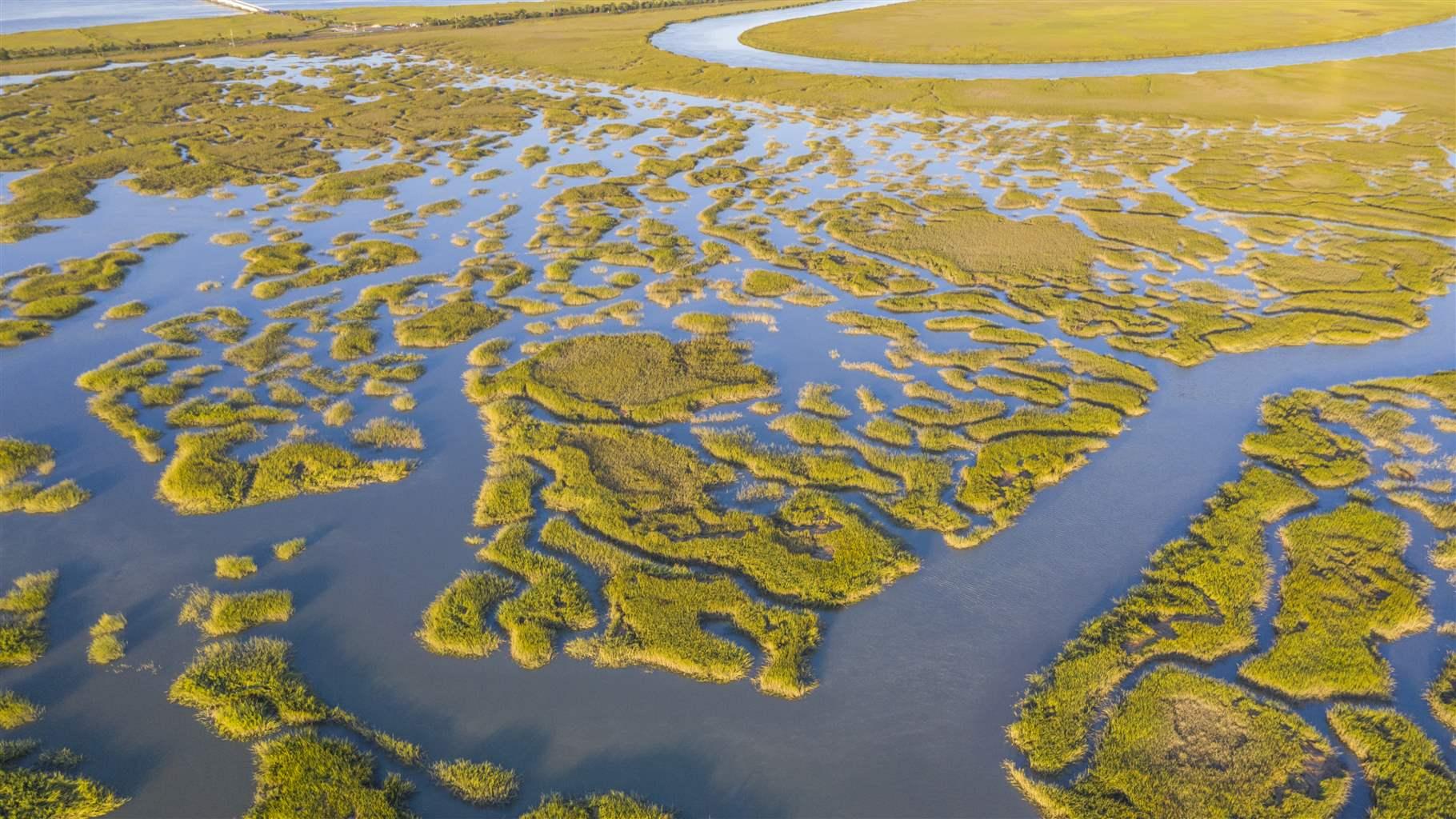This aerial photograph captures a vibrant wetland landscape reminiscent of the Everglades. The scene is dotted with numerous small islands and landmasses, painted in varying shades of yellowish-green foliage, likely influenced by the time of day the picture was taken. These islands are interspersed throughout a network of clear, shallow blue water, creating a patchwork of land and water. Small rivers and creeks meander through the terrain, adding to the intricate layout. In the background, the landscape transitions to a more solid golden-brown land, featuring a distinctive U-shaped river that courses through the area. This photograph showcases the intricate and dynamic beauty of this marshland ecosystem, with its mixture of water, vegetation, and changing terrains.